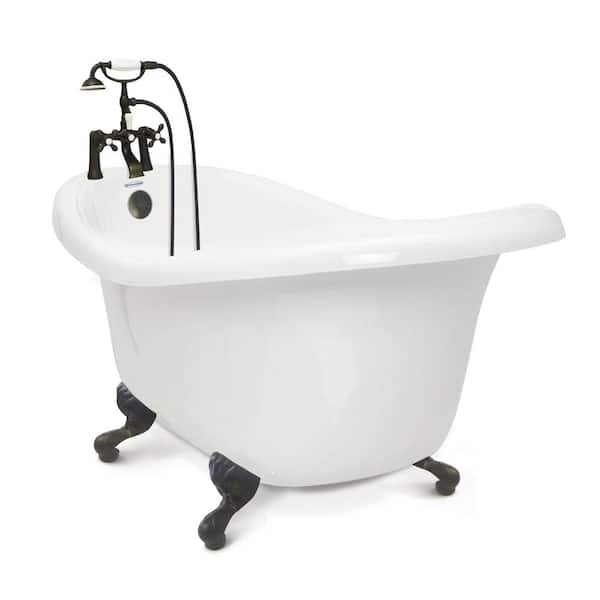This image features a white, unusually shaped clawfoot bathtub set against a plain white background. The tub elegantly curves upward towards the back, creating a wavy top design. It rests on four black, curved feet, with three visible in the photo and the fourth implied. The clawfoot design has an old-fashioned appeal, possibly wrought iron or cast iron. 

At the rear of the tub, the faucet hardware includes a vintage-style, gray to black metal or steel fixture with separate hot and cold handles, and a central lever that switches water flow between the tub faucet and a connected handheld shower head. The handheld shower head, resembling a round spaceship, is attached by a flexible hose. Additionally, there is an overflow drain, round and gray, situated near the top to prevent water overflow. The bathtub, likely photographed for an advertisement, is depicted diagonally, emphasizing its depth and unique design elements.